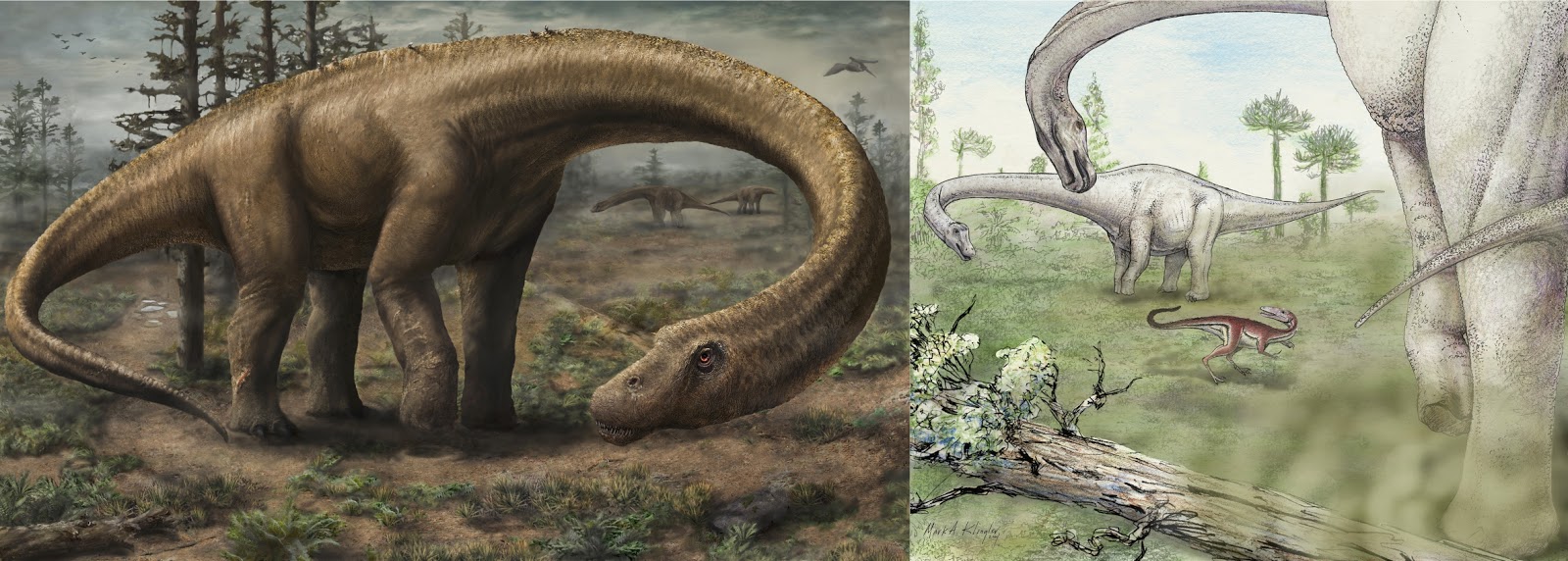The artwork features two side-by-side images depicting dinosaurs in different environments. The left image showcases a large, bronze-colored dinosaur with a long neck and tail, set against a dark, gloomy forest with sparse, naked trees and patchy grass. Additional dinosaurs can be seen in the background. The right image contrasts sharply, displaying three dinosaurs with long necks, primarily gray in color, and a small, dark brown dinosaur running between them. This scene is brighter, featuring a light blue sky, more vibrant grass, and scattered trees, with a fallen tree in the foreground.